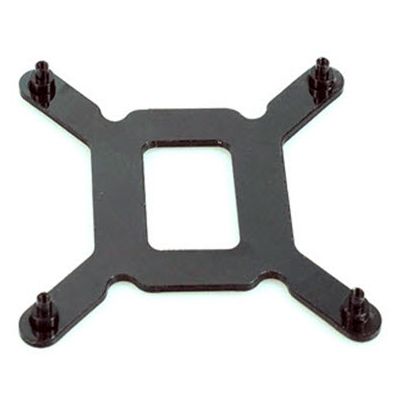This photograph features a matte black metal TV mounting bracket against a clean white background. The central portion of the bracket is a rectangular cutout, creating an O-shaped block. This bracket design includes four appendages extending diagonally from each corner of the rectangle. Each of these arms ends in a rounded leg, equipped with a black nut and protruding thick black screw, signaling the points where the mount attaches to its respective surface or equipment. The metal of the bracket is visibly thick, with subtle reflections seen within the cutout area, indicating its solid manufacturing. The context suggests this could be a component from an instruction manual or guide, intended for securely mounting a flat-screen TV to a wall.